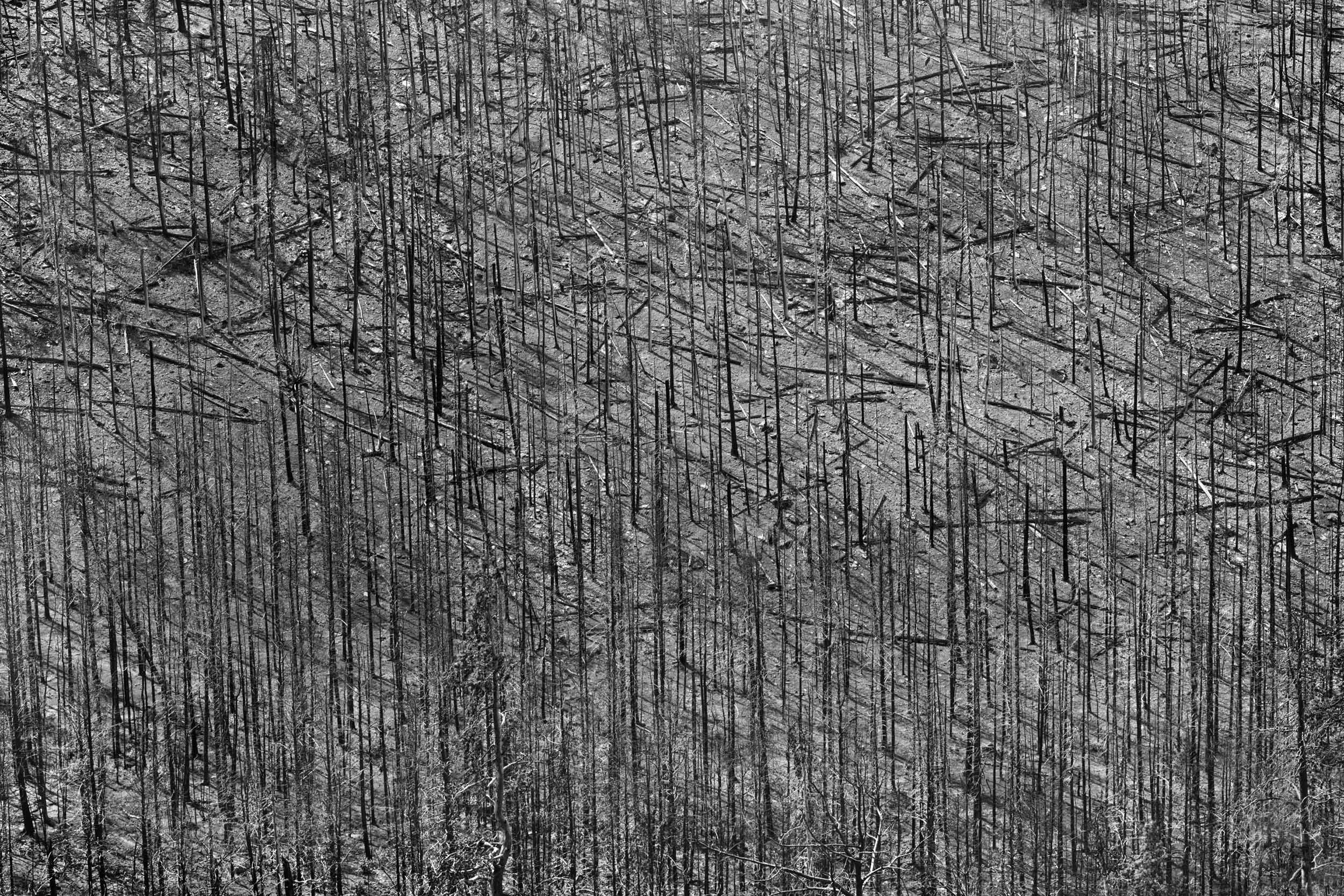The image features a light gray background covered with a myriad of dark gray, pin-like, horizontal and vertical scribbles reminiscent of an abstract drawing or illustration. This black-and-white scene elicits the illusion of a forest devoid of leaves, where intricate, overlapping lines suggest both dense and sparse tree areas. In the bottom portion, the scribbles define the faint outlines of trees, some appearing as if they've been covered in snow. The top section, dominated by more chaotic and darker strokes, hints at an area where trees may have fallen, possibly due to deforestation or a fire. This rectangle image, striking in its complexity and stark contrast, manages to evoke a sense of devastation while also being visually captivating and thought-provoking.